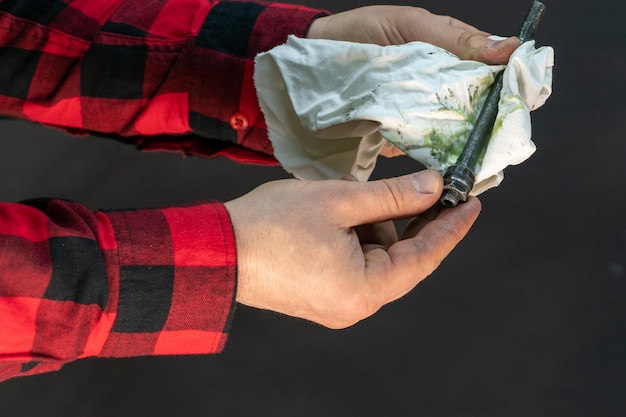The photograph captures a vivid, up-close image of a Caucasian male's hands and forearms, clothed in a long-sleeved red and black plaid flannel shirt, engaged in cleaning a long, metal bolt. The hands are positioned horizontally across the frame, holding a white rag stained with green grease, indicative of the man wiping off oil and grime from the dark, approximately six to eight-inch long bolt. The detailed shot, set against a black background, focuses exclusively on the hands and the task, emphasizing the meticulous action of cleaning the machinery part, possibly for automotive or industrial use.